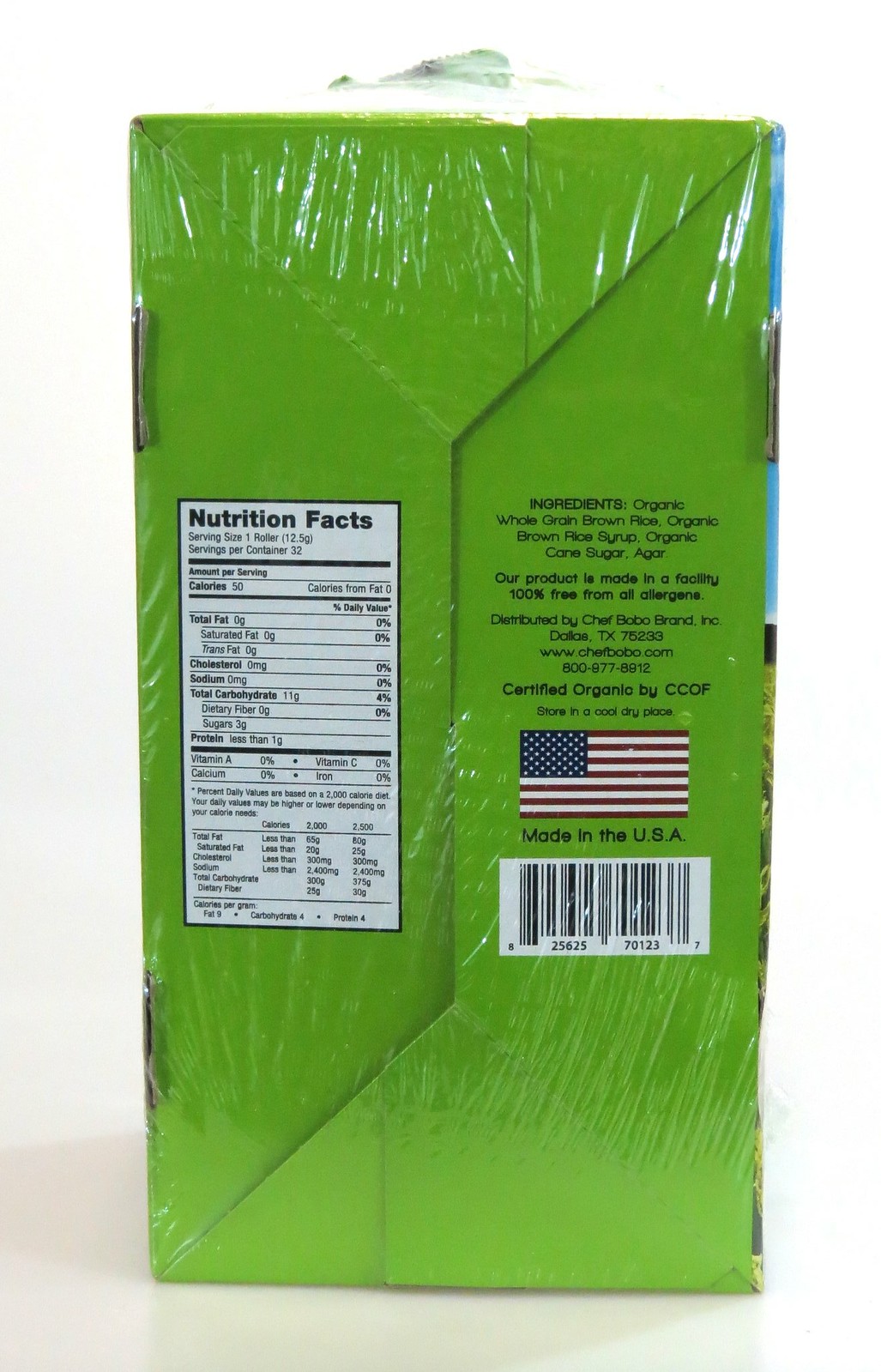This image captures the back of a food product packaging, predominantly showcased in a vibrant green color. The packaging features a prominently displayed nutrition facts label and a comprehensive list of ingredients. The nutrition facts section indicates that the serving size is one roller, with a total of 32 servings per container. Each serving contains 50 calories, 0 grams of fat, 11 grams of carbohydrates, and 1 gram of protein. The nutrition facts also reveal that the product contains no cholesterol, sodium, dietary fiber, vitamin A, vitamin C, calcium, or iron, with each of these showing 0% of the daily value. The ingredients listed are whole grain brown rice, organic brown rice syrup, organic cane sugar, and agar, indicating a focus on organic and whole grain components.